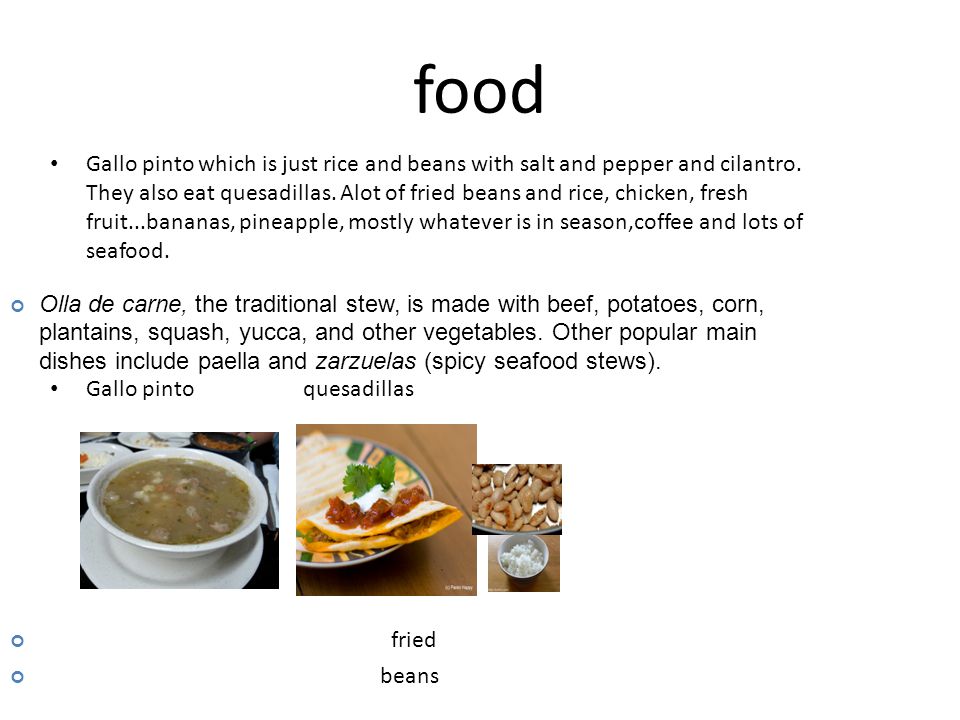The image appears to be a simplistic, black-and-white PowerPoint slide with the title "Food" prominently displayed at the top. The slide includes a series of bullet points detailing various traditional dishes. The first bullet point mentions "gallo pinto," which is described as rice and beans seasoned with salt, pepper, and cilantro. Subsequent bullet points list other foods such as quesadillas, fried beans and rice, chicken, various fresh fruits like bananas and pineapples, seafood, and coffee. Additionally, it describes "olla de carne," a traditional stew made with beef, potatoes, corn, plantains, squash, yucca, and other vegetables, as well as other dishes such as paella and zarzuela, which are spicy seafood stews. Below the text, a series of images illustrate the foods mentioned: a white bowl of soup on a saucer, a soft-shell taco or quesadilla topped with salsa and cream, and small plates displaying fried beans and rice. The overall design is very basic, lacking any elaborate design elements or color beyond black text on a white background. The slide breaks the general PowerPoint guideline by including extensive text in bullet points, which ideally should be concise.